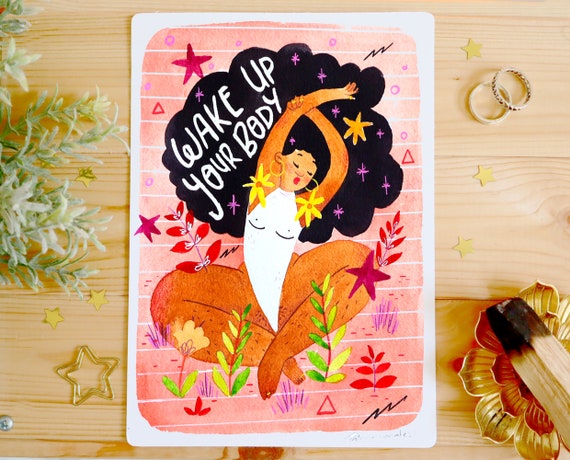The image captures a contemporary and whimsical artwork displayed on a light wooden desktop. The wooden surface has a rustic feel, enhanced by visible grains, lines, and knots. To the left, pale green plants are peeking into the scene, while the bottom-right corner features a tray with recently burned Palo Santo. Two rings are situated in the upper-right corner, and gold star outlines and confetti are scattered around.

The centerpiece of the image is a vibrant poster with a white border and a pink background adorned with white stripes. Dominating the poster is an illustration of a dark-skinned woman, who is sitting cross-legged as if meditating, with her arms outstretched and bent as though she is stretching. She is portrayed wearing a white leotard, and her strikingly large and poofy black afro, embellished with purple stars and looking almost like a galaxy, forms a halo around her. Inside her afro is the white text, "Wake up your body." 

Adjacent to her, sunflowers serve as her hoop earrings, and flowers of varied colors—red, green, and purple—along with leaves and starfish, further enrich the scene. The background, blending shades of pink, completes the image's enchanting and dreamy atmosphere.